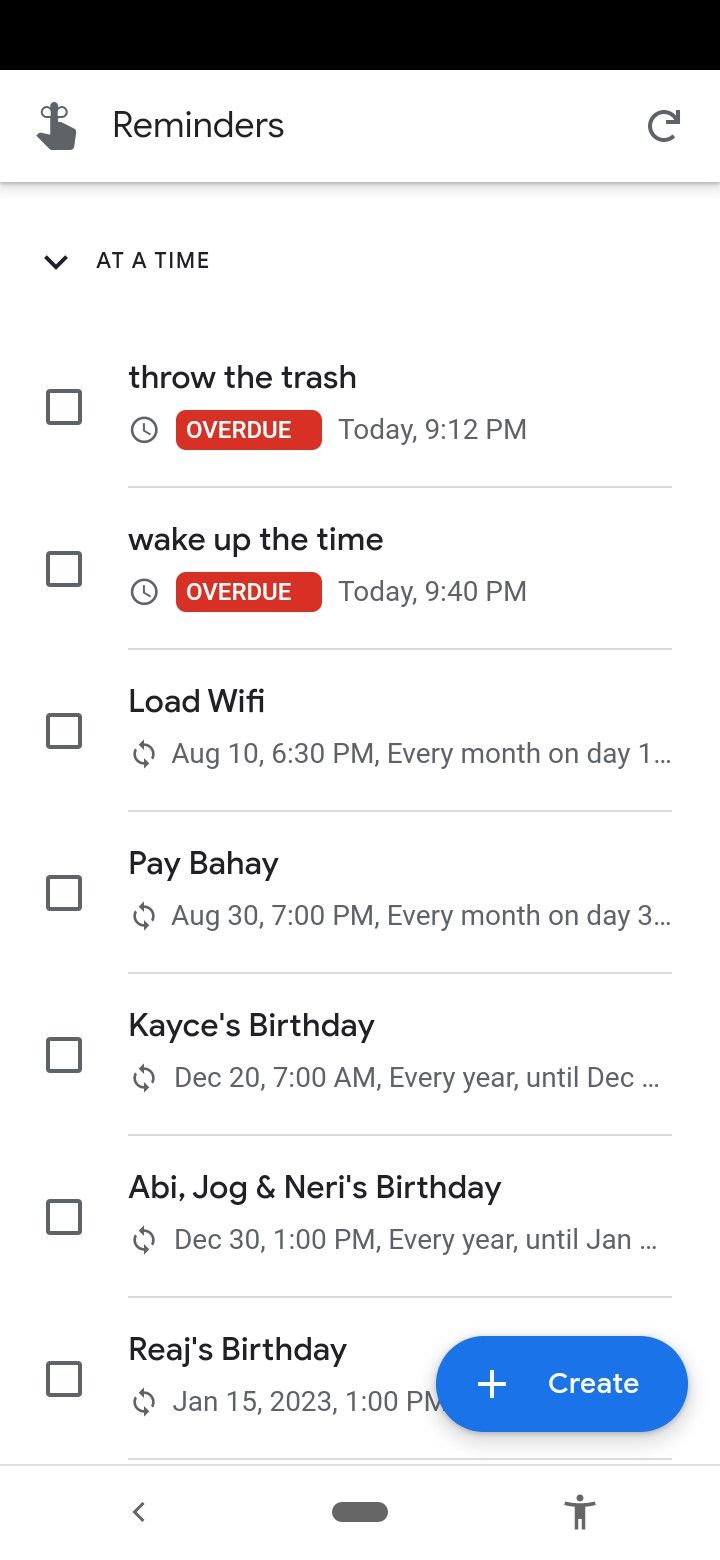This is a detailed descriptive caption for the provided image:

---

The screenshot is taken from a smartphone, displaying a reminder application. At the top, there is a black bar spanning the entire width of the screen. Below the bar, an icon of a finger with a string tied around it appears, labeled "Reminders." On the right-hand side of this section, there is a refresh icon for reloading the page. 

Below this, there is an option labeled "Add a Time." The main area of the screen lists several reminders, each with a checkbox beside it. The items are as follows:

1. **Throw the Trash** - Marked as overdue, with a due time of today at 9:12 p.m.
2. **Wake Up the Time** - Also overdue, with a due time of today at 9:40 p.m.
3. **Load Wi-Fi** - Scheduled for August 10th at 6:30 p.m., recurring every month on the 1st.
4. **Pay Bahay** - Scheduled for August 30th at 7:00 p.m., recurring every month on the 3rd.
5. **Kacey's Birthday** - Scheduled for December 20th at 7:00 a.m., recurring annually.
6. **Abby Joganeri's Birthday** - Scheduled for December 30th at 1:00 p.m., recurring annually.
7. **Rea's Birthday** - Scheduled for January 15th.

To the right of these items, there is a blue oval button with a plus sign in the center, labeled "Create." 

---

This description provides a detailed and structured overview of the screenshot content.